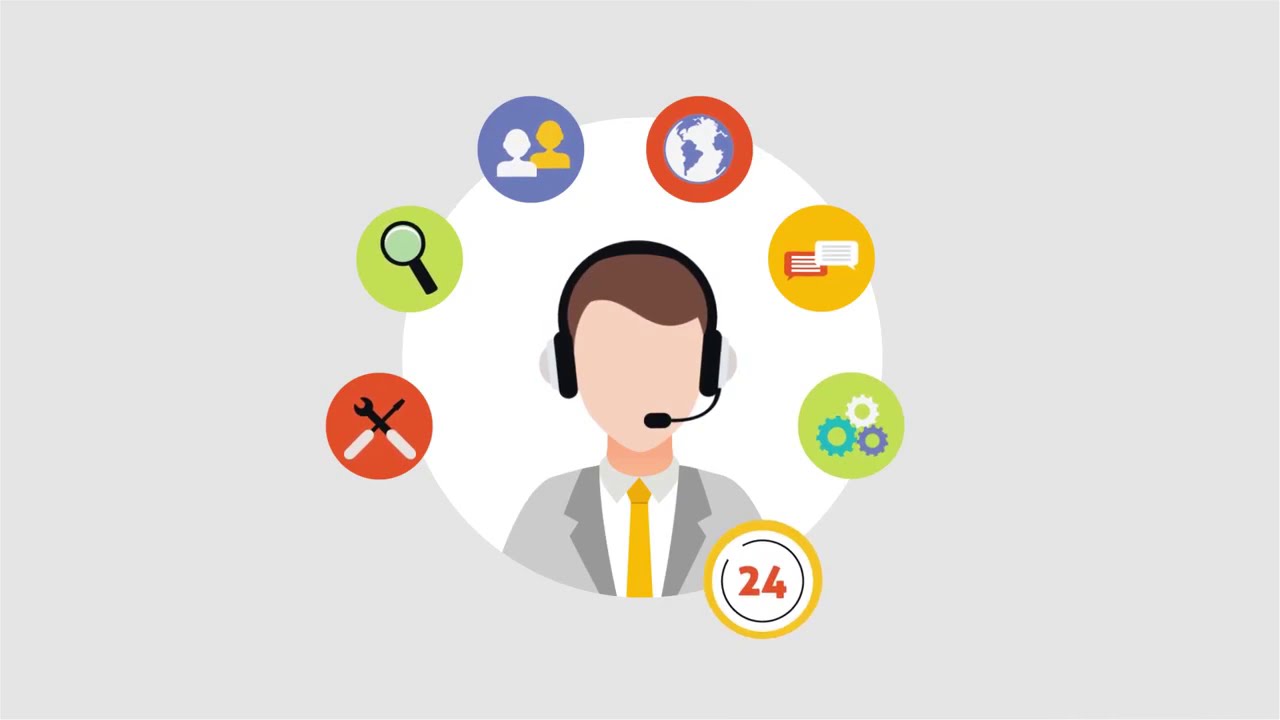The image features a stylized, faceless customer service representative positioned centrally within a white circle against an off-white, beige background. He wears over-the-head headphones with a microphone, partnered with a white collared shirt, a yellow tie, and a gray suit jacket. His hair is brown, parted to the side. Around the edge of the white circle are seven smaller, color-coded circles, each containing unique symbols. These include a red circle with a screwdriver and wrench, a lime circle with a black magnifying glass, a blue circle with two white and orange heads, a red circle with a blue and white globe, an orange circle with two text message rectangles, a lime circle with three gears, and another circle with red text displaying "24". The scene is set against a gray background, and the overall image is wider than it is tall, resembling the shape of a high-definition television. The colors featured within the image include various shades of yellow, gold, red, purple, blue, and green, suggesting that it's likely an advertisement or logo without additional text or context.